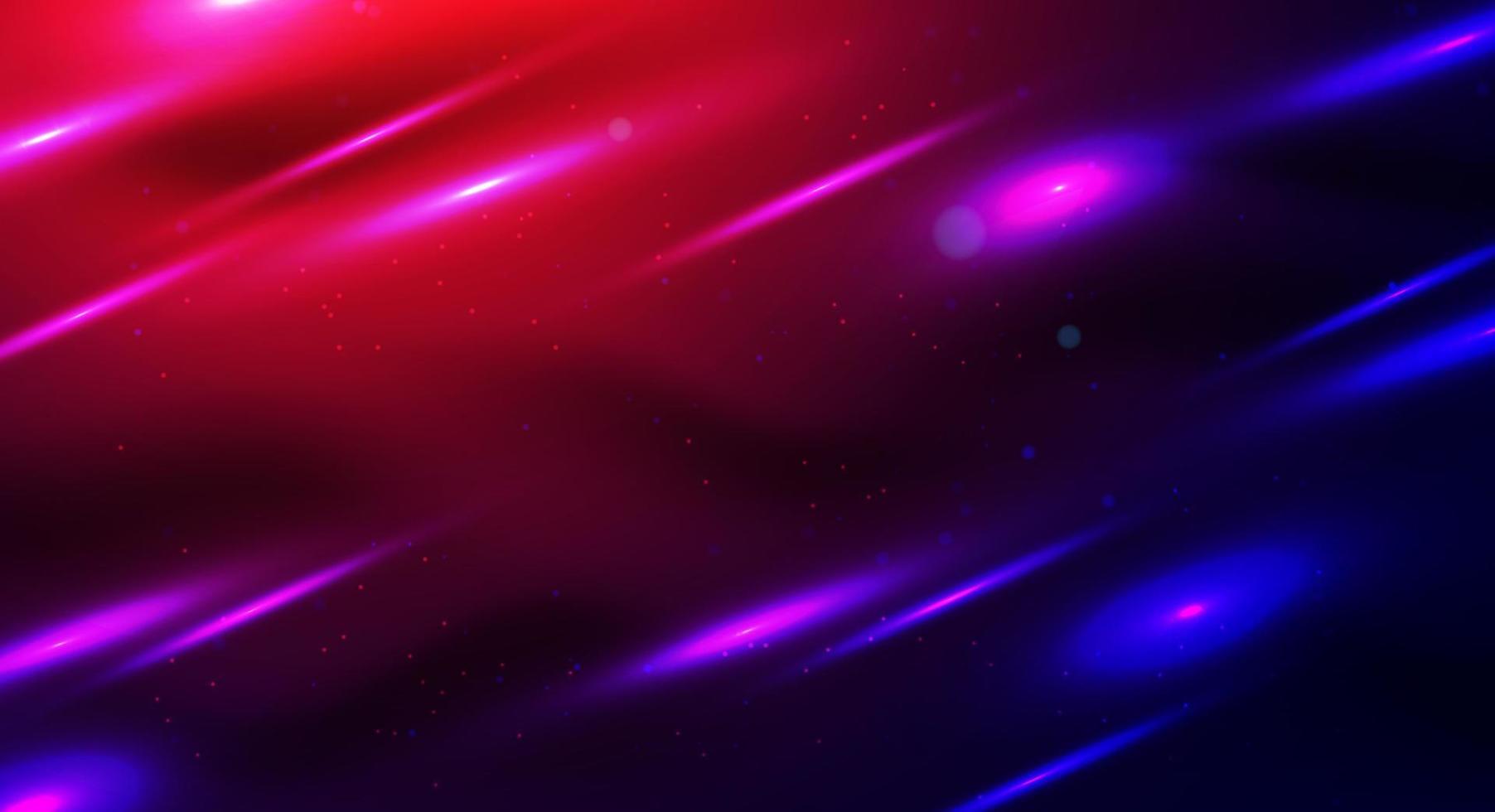This abstract digital artwork prominently features a diagonal composition that divides the image into distinct color zones. In the top left corner, a fiery red background is interspersed with vibrant pink streaks and dotted with white specks tinged with pink. These radiant streaks evolve into deep purple as they traverse diagonally downward, merging into a darker palette. As the background shifts from dark blue to a nearly black hue towards the bottom right, the pink and purple streaks transform into luminous blue lines with pinkish-purple centers. The artwork displays a dynamic gradient of colors, from the red and purple in the upper sections to the dark blue and black below. Throughout the piece, numerous small dots—some illuminated in shades of red, UV, and dark blue—create an ethereal star-like effect. Certain larger dots have glowing rings around them, adding depth and a cosmic feel to this vividly detailed composition.